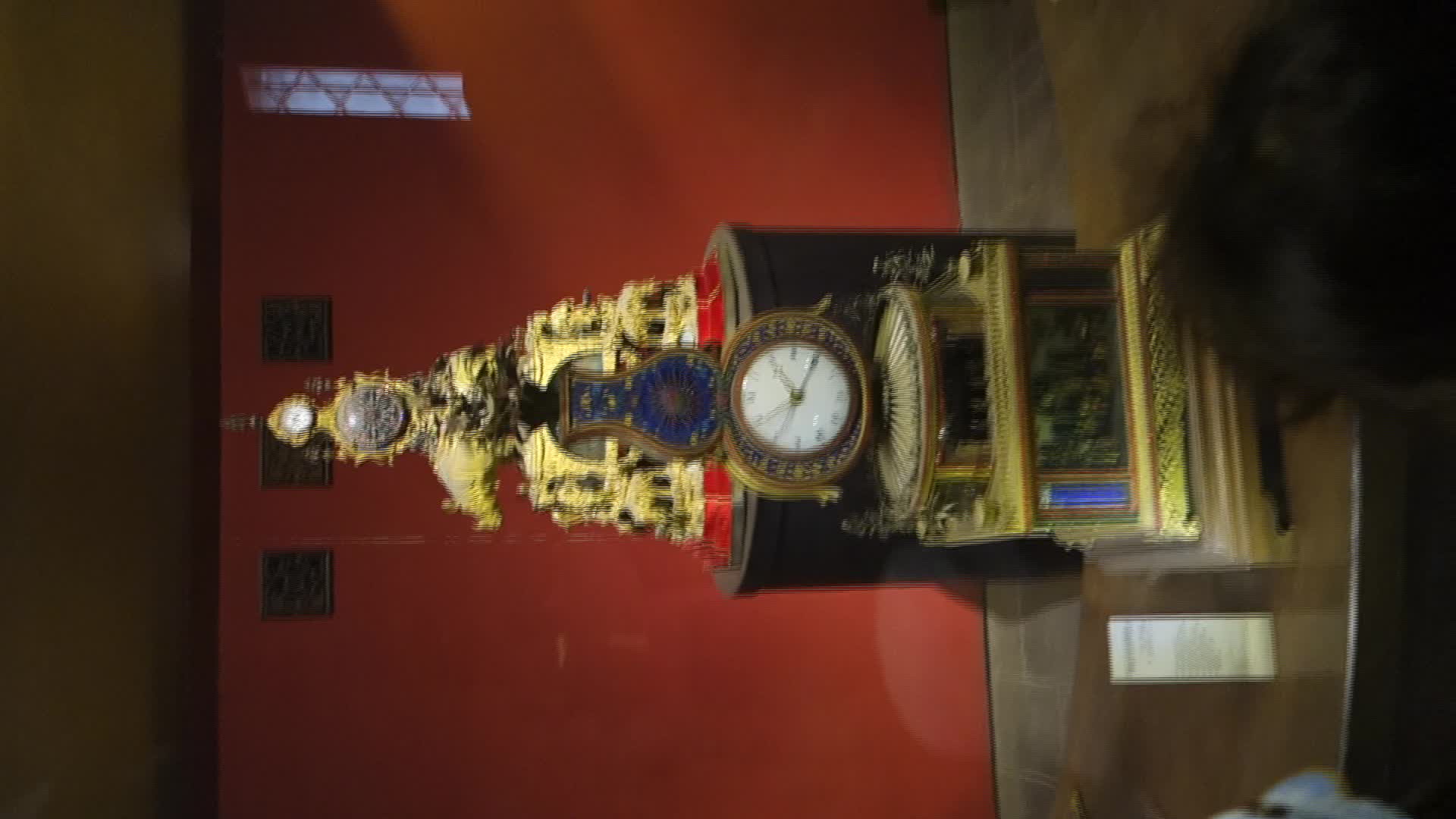The image captures an intricately designed, ornate clock that has been rotated 90 degrees to the left, making the top of the clock point towards the left side of the photo. The clock exhibits a striking, architectural aesthetic reminiscent of ancient Indian or Thai craftsmanship, featuring elements like a steeple and detailed ornamentation. The base of the clock is gold, followed by a black section in the middle, above which more gold leads into a temple-like structure. The clock face is completely white, adorned with gold hour and minute hands, and surrounded by a golden frame. There are also purple and black jewels embedded in the design, adding to its regal appearance. The clock rests on a brown surface with a red wall backdrop, suggesting it is displayed in a museum. A white placard is visible to the left of the clock, likely providing information about the exhibit, though its text is unreadable due to the image's orientation. In the background, there are blurry figures and possibly another ornate statue, enhancing the museum-like setting.